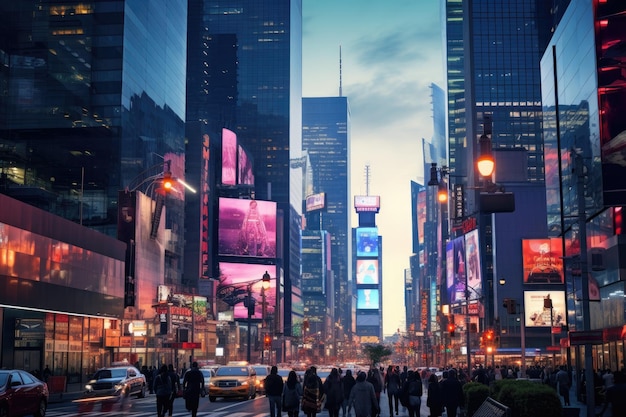The image captures a bustling cityscape at dusk or early evening, characterized by a dramatic skyline of towering skyscrapers lining both sides of the photo. The sky, painted in twilight shades of pink, orange, blue, and red, suggests a cloudy day with the sun setting. The streets below are alive with activity: illuminated billboards and electronic advertisements form a vibrant row in the distance, casting colorful reflections onto the scene. In the front center, silhouettes of people walk down a wide sidewalk, their figures blurred in motion amid the city's hustle and bustle. To their left, yellow cabs and other cars navigate the road, with streetlights glowing warmly on both sides. The overall scene embodies the dynamic and energetic spirit of a major downtown area, reminiscent of cities like New York.